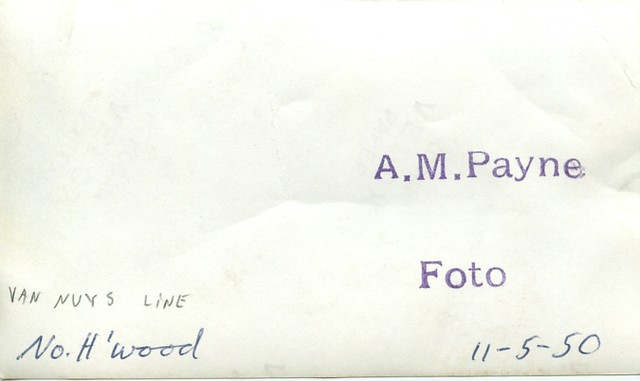The image depicts a horizontally rectangular envelope against a white background. On the front of the envelope, in the right half centered, there is a stamped mark reading "A. M. Payne" followed by "photo" in a stylized "FOTO" format. Below this stamp, the date "11-5-50" is clearly printed, indicating November 5th, 1950. In the bottom left-hand corner, written in a pen differing in color—black for "Van Nuys Line" and blue for "No H-Wood"—there's an address, suggesting a connection to someone in North Hollywood. There is no postage stamp or postmark on the envelope, indicating it wasn't sent via mail and may have been kept for record-keeping or was intended to be sent and never was.